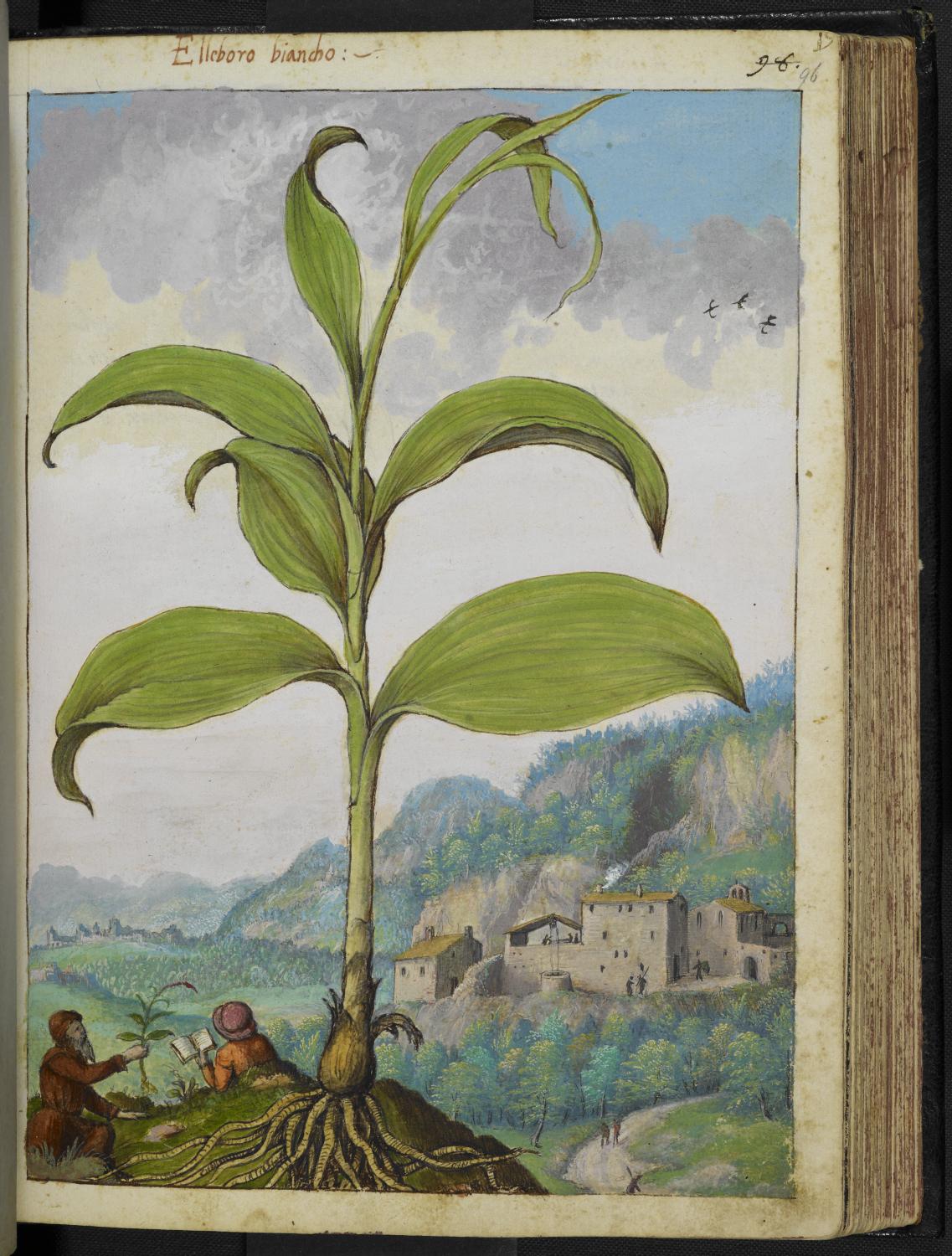This vivid illustration, appearing like a page from an old storybook, captures a whimsical scene reminiscent of a fairy tale such as "Jack and the Beanstalk." The open book reveals the handwritten words "Elaboro Biancho" at the top of the right-hand page, with the numeral 96 in the upper right corner outside the image border. The central focus is a colossal plant with large green leaves and a bulbous root system extending from its base, portraying an exaggeratedly grand scale. Near the base of this towering plant, an elderly man is seen holding a smaller stalk, accompanied by a child who is absorbed in reading a book. Their diminutive figures emphasize the plant’s enormous size, which dominates three-quarters of the page. The background features a picturesque landscape with a blue, cloudy sky, rolling hills, and a large house or cluster of stone houses that resemble a medieval town, complete with archways and an open-air well. Trees and additional hills enhance the serene, storybook quality of the setting.